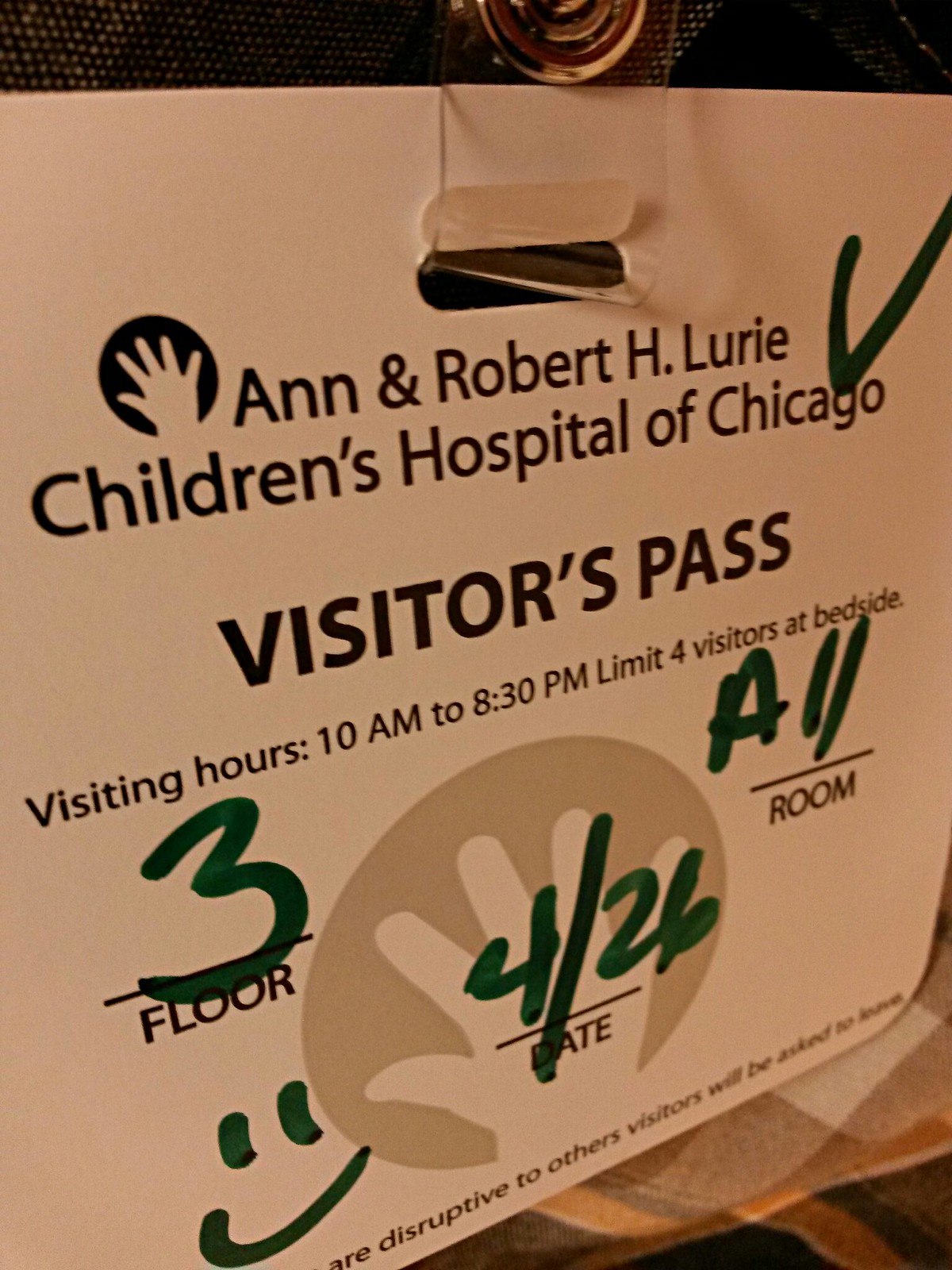The image depicts a visitor's pass for the Ann and Robert H. Lurie Children's Hospital of Chicago. The pass is white, with black text and features a prominent round black circle with a white hand in the middle, serving as a logo at the top. Below the logo, it states "Ann and Robert H. Lurie Children's Hospital of Chicago" and "Visitor's Pass." The pass details the visiting hours as 10 a.m. to 8:30 p.m. and mentions a limit of four visitors at the bedside. It provides specific information such as the floor (3), room number (A11), and the date (4-26). This information is written in green ink, and there is a green marker check mark in the top right corner alongside a green smiley face at the bottom left. Additionally, there's some unreadable small text at the very bottom of the pass. The pass appears to be clipped to someone's clothing, possibly attached via a button or similar device.